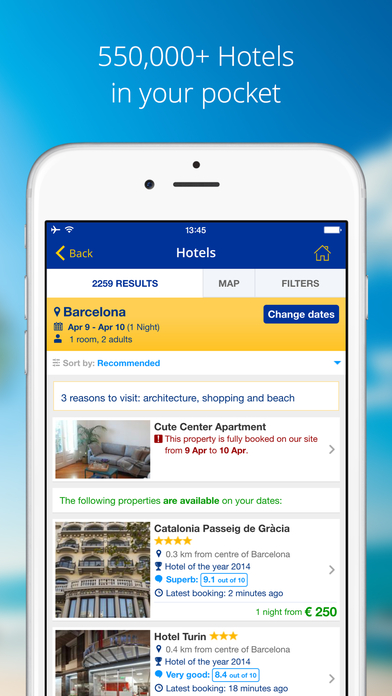Screenshot of a vibrant blue advertisement featuring a smartphone display advertising hotel options. The top portion of the image has a sky-blue background with the text "5,500,000 hotels in your pocket" in bold white font. Below this text, a graphic of a white smartphone with white bezels is prominently displayed. 

On the smartphone screen, details are meticulously depicted:
- A blue notification bar at the top shows icons for full Wi-Fi signal, airplane mode activated, the time as 13:45, and a full battery.
- Below the bar, a back button is visible.
- Central to the screen is the word "Hotels" in white font.
- Further down, a home button is located for easy navigation.
- A white rectangle below displays "2,259 results."
- Following this, two gray buttons are featured: one labeled "Map" in red font, and another labeled "Filters," also in red font.
- Below the buttons, a yellow rectangle with blue font reads "Barcelona," accompanied by the information "April 9th to April 10th, one night, one room, two adults." Adjacent to this, a clickable option says "Change dates."
- At the bottom, a white rectangle indicates "Sort by recommended."
- Closing the presentation, the text "Three reasons to visit: architecture, shopping, beach" provides compelling incentives.

This detailed interface suggests a user-friendly tool for finding the perfect hotel among a vast selection, with specific features to tailor the search experience.